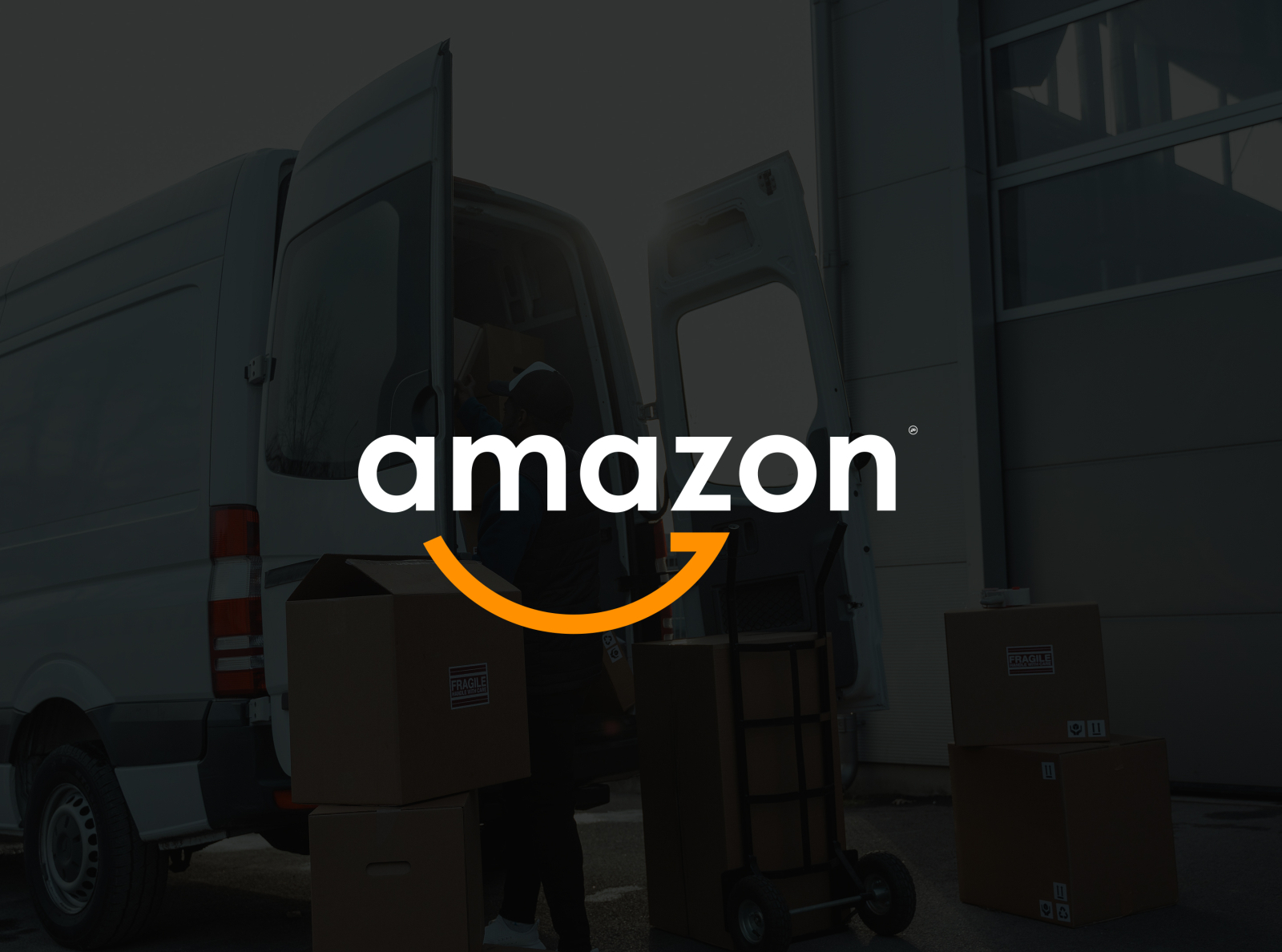The image captures a single screenshot featuring the iconic Amazon branding. Dominating the center of the screen are the words "Amazon" rendered in bright white lowercase letters. Beneath the text, a yellow line arcs in a subtle smile-like shape, deviating from Amazon's typical logo but still recognizable as a variant. 

In the background, a faint and somewhat blurry scene unfolds. It depicts a white panel van with its rear doors open, revealing a person loading boxes into the vehicle. Beside the person stands a two-wheel cart, which supports a larger box. Scattered around are several other boxes, some adorned with fragile stickers. One box is partially opened, while another one sits nearby, hinting at an organized but busy dispatch operation outside what appears to be a storage facility. Despite the blurry nature of the background, it seems to be a sunny day. The boxes, many of which feature prominent white labels, add to the sense of a bustling, logistical setting.